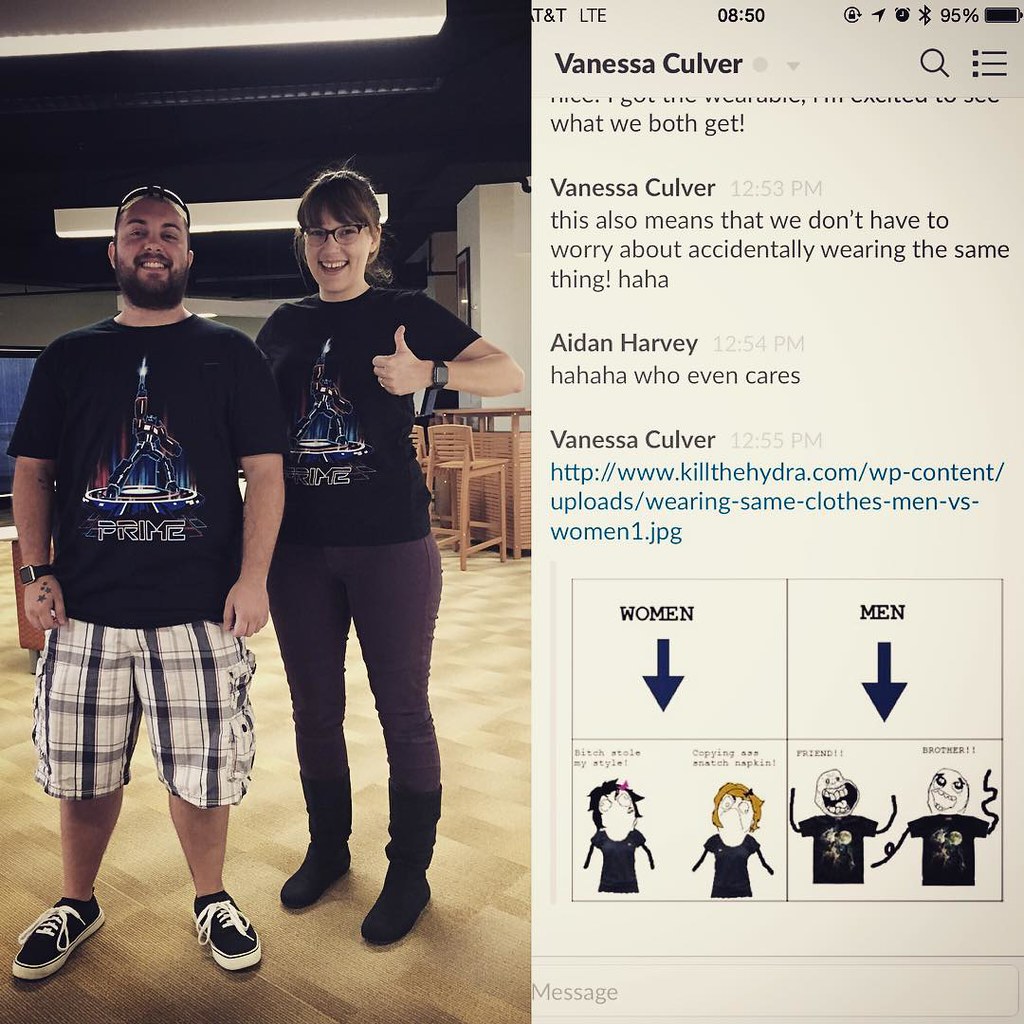In this composite image, the left half features a photograph of a man and woman, identified as Aiden Harvey and Vanessa Kolber, respectively, dressed in matching black t-shirts emblazoned with an Optimus Prime design. Aiden, standing on the left, sports glasses on his forehead, a beard, and wears white and black checkered pants paired with black sneakers adorned with white laces. Vanessa, standing on the right with her hair pulled back and sporting bangs, wears glasses, black pants, black boots, and a smartwatch on her left wrist, which she uses to give a big thumbs up. They are indoors, with a carpeted floor, wood furniture, some chairs, and a bar visible in the background. The right half of the image shows a screenshot from a phone depicting a conversation between Vanessa and Aiden, including text messages with timestamps, a hyperlink, and a meme reflecting on the humor of accidentally wearing matching clothes.